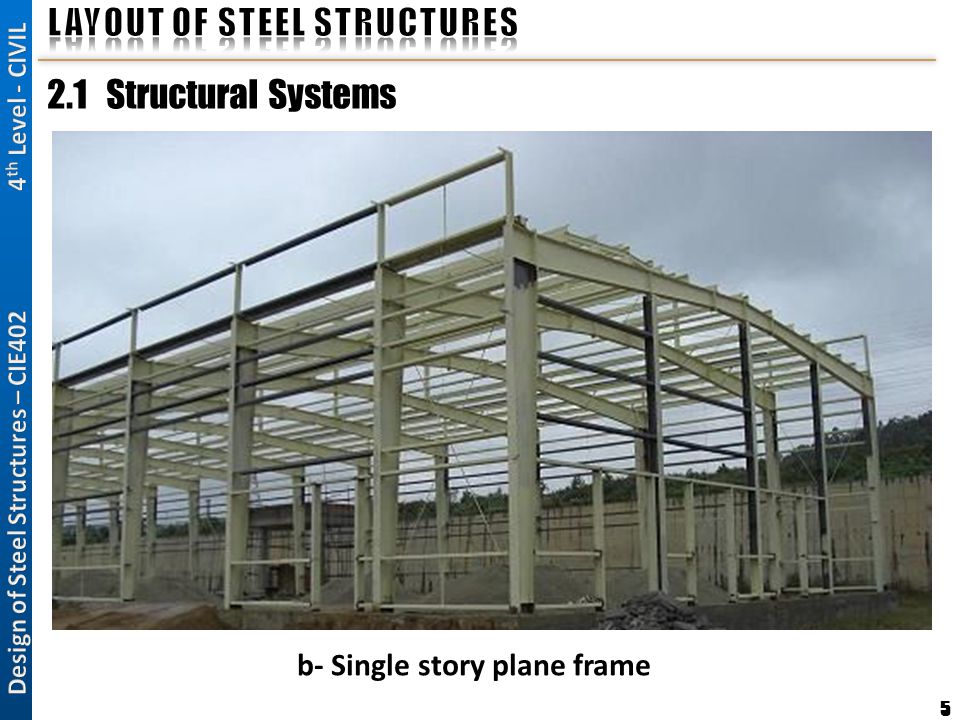This image features the open framework of a substantial steel structure, approximately 30 to 50 feet tall, set against a cloudy, gray sky. The structure, made entirely of metal beams, stands centered in a field with a wooden fence and a tree line visible at the bottom. The structure is beige in color, contributing to the muted palette of grays, tans, blacks, browns, and a hint of green in the surrounding vegetation.

Text overlays play a significant role in this composition. At the top, in black, are the words "Layout of Steel Structures," followed by "2.1 Structural Systems" in bold type. A prominent blue vertical stripe along the left side contains white text that reads "Design of Steel Structures, CIE 402, Fourth Level, Civil." Below the photograph, also in black, is the caption "B - Single Story Plain Frame."

This image appears to serve an educational purpose, likely in the context of architectural or civil engineering studies, illustrating a single-story plain frame steel structure.